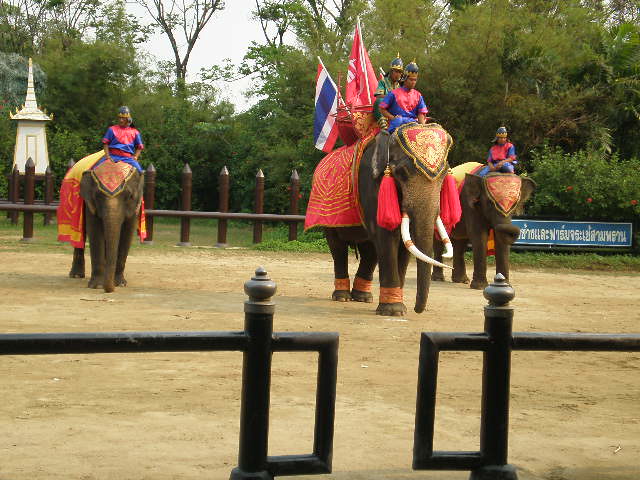The image depicts three ornately decorated elephants in a Southeast Asian setting, most likely Thailand, as evidenced by the presence of the Thai flag. The scene is viewed from behind a brass rectangular barrier attached to two spokes, looking into a dirt enclosure. The elephants, positioned in a line with the middle one being the closest and largest, are adorned with elaborate red garb that includes red tassels hanging from their ears and red blankets draped across their bodies. Their heads feature decorations resembling red shields with gold designs.

The middle elephant stands out with its two large tusks and two riders: the front rider in a blue and red outfit, and the rear rider in an emerald green outfit with a metal helmet. This elephant also displays two flags on its back: the Thai flag with red, white, and blue stripes, and a red flag with an indeterminate design, possibly the Hong Kong flag.

The other two elephants each have a single rider. The rider on the left elephant wears a blue and red top paired with a round helmet, while the rider on the right elephant dons a similar uniform complete with a helmet. In the background, there is a wooden stake post fence, a blue sign with white Thai writing, a white pagoda to the far left, a grassy area, and a variety of tall green trees. This richly detailed scene highlights both the cultural elements and the majestic appearance of the elephants and their riders.